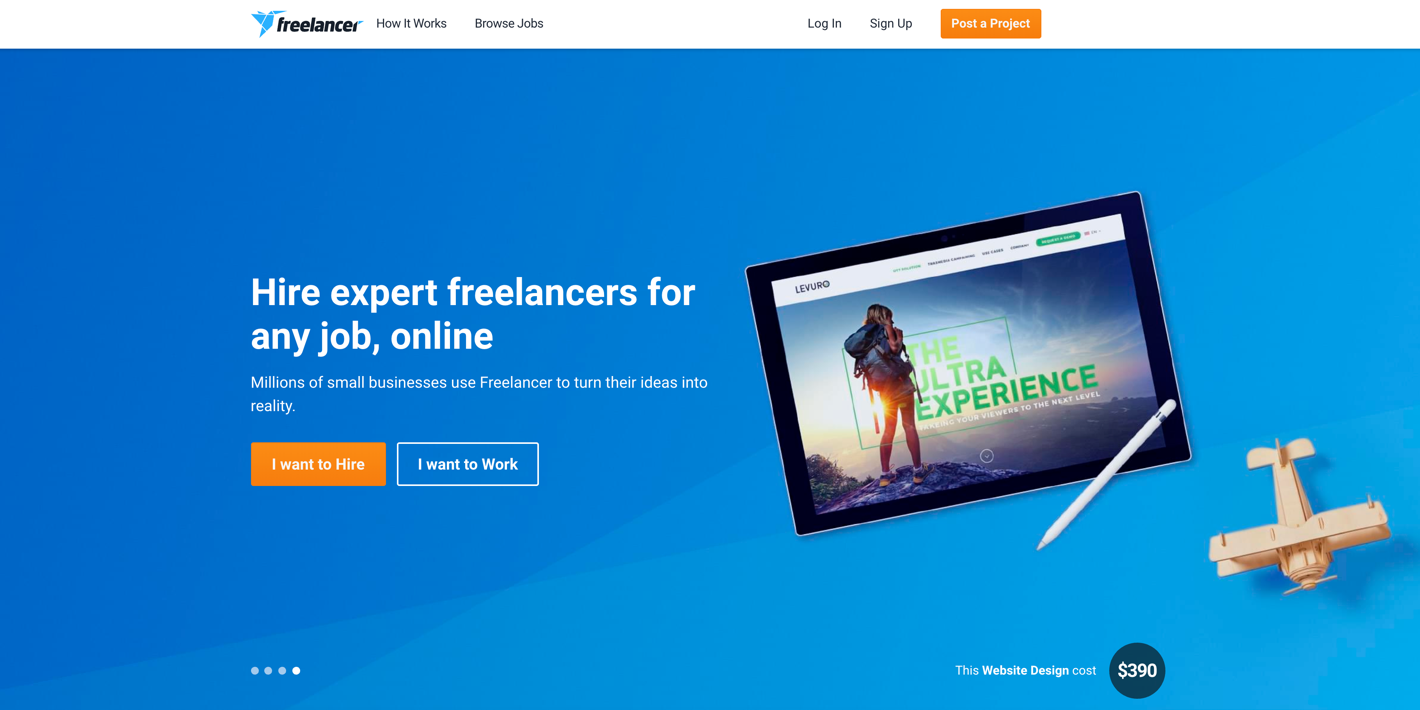This image is a snapshot of the Freelancer website, showcasing its user interface. At the top-left corner, an artistic representation resembling a hummingbird crafted from folded paper, likely computer-generated, bears the text "How it works: Browse Jobs." Above this, navigation options for "Log In" and "Sign Up" are displayed. 

An orange button labeled "Post a Project" prominently stands out. Below, the webpage is adorned with a gradient background transitioning from a deep royal blue on the left to a lighter shade on the right, especially brightening at the bottom-right corner.

In the background, a digital tablet is visible with the branding "Levero," spelled out in large white letters, promoting "The Ultra Experience." The phrase "Take your view to the next level" is partially discernible. Adding to the tech-themed design is the illustration of a computer pen.

The headline reads "Hire expert freelancers for any job online," followed by a subtext stating, "Millions of small businesses use Freelancer to turn their ideas into reality." Two call-to-action buttons are included: an orange button labeled "I want to hire" and a blue button labeled "I want to work." The overall aesthetic is modern and professional, emphasizing convenience and accessibility for both employers and freelancers.